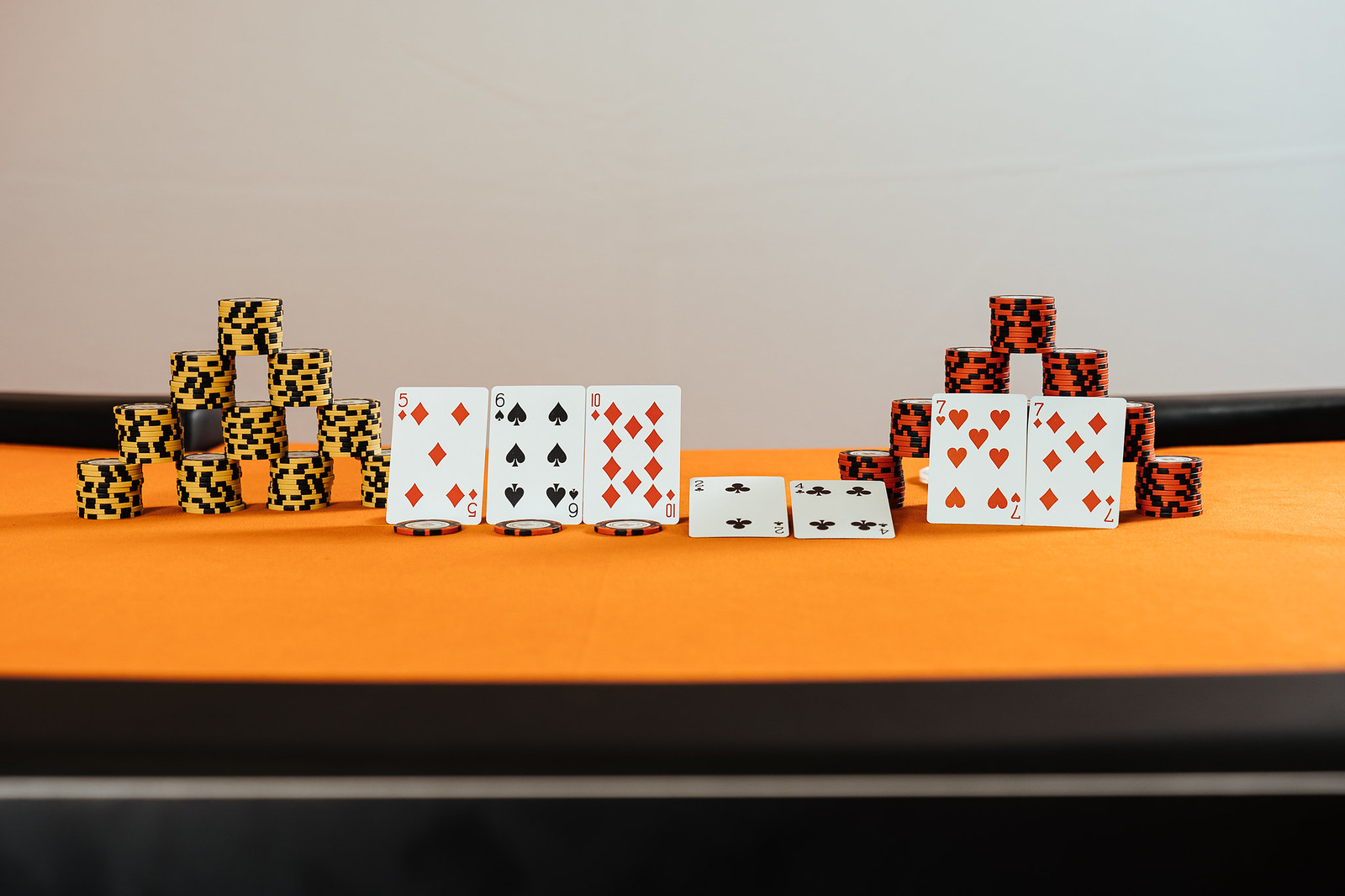In this photograph, an elaborate setup is displayed on an orange surface, though it is unclear whether this is a blanket or a countertop. The image's foreground is out of focus, with the photographer’s emphasis on the central objects creating a depth-of-field effect. A blurred black section with a horizontal gray line runs along the bottom, followed by the indistinct border of the orange surface.

The focal point is a meticulously arranged collection of poker chips and playing cards. In the center, stacks of poker chips create symmetrical pyramid structures. On the left, yellow and black poker chips form a detailed tower: four equal-height stacks at the base, three bridging stacks above, followed by layers of two chips, and then one chip on top to complete the pyramid. Propped up by these stacks are a five of diamonds, a six of spades, and an eight of diamonds. Additionally, a two of clubs and a four of clubs lie flatter on the surface.

To the right, an identical pyramid of red and black poker chips mirrors the arrangement on the left. Leaning against this structure are a seven of diamonds and a seven of hearts. The backdrop consists of a blurry edge transitioning into a light gray wall, likely influenced by the lighting conditions. This setup suggests a poker table setting, albeit with an unconventional orange surface.